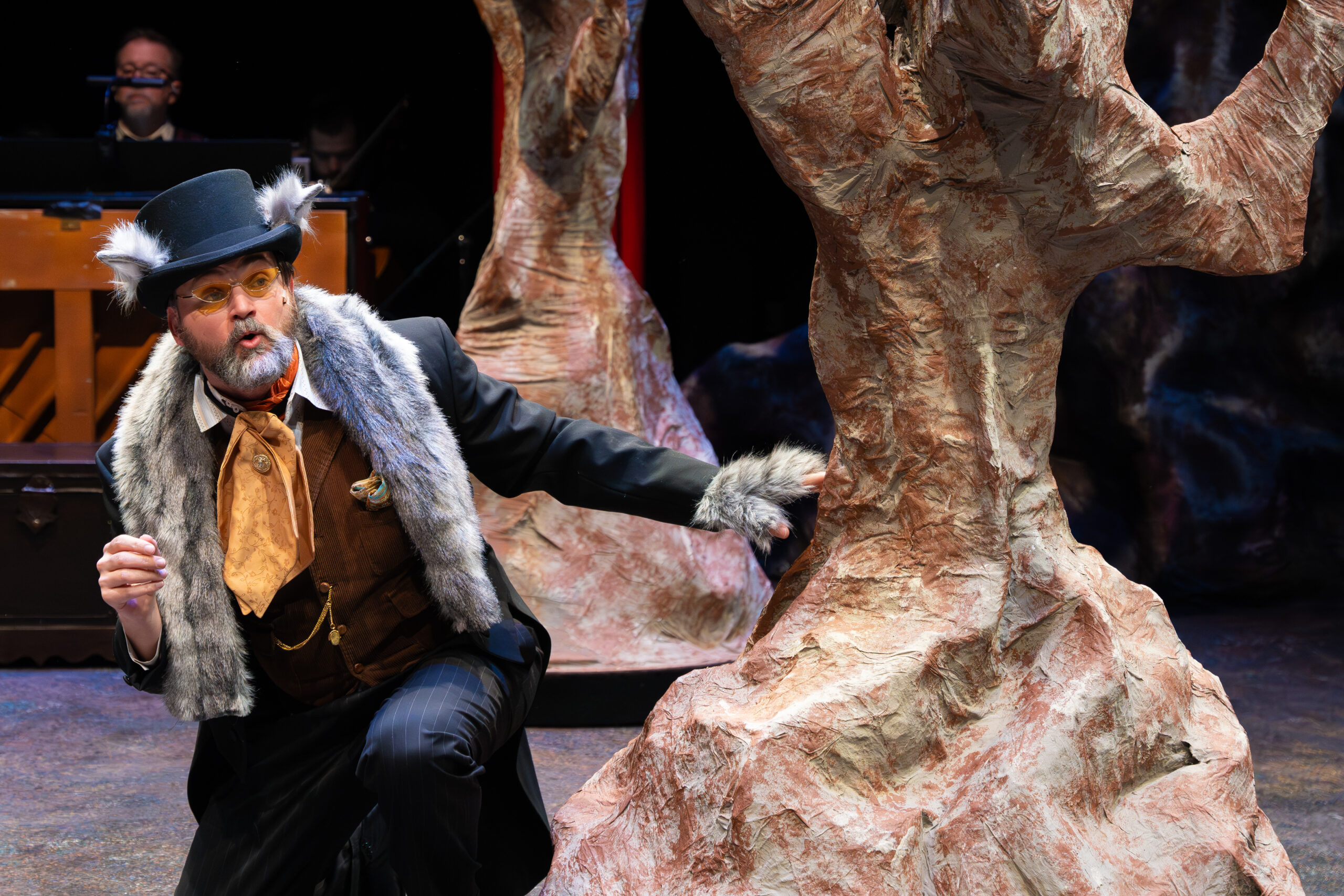The image captures a vividly detailed stage performance in a color landscape photograph. The central figure, positioned on the left side of the scene, is an actor adorned in an elaborate, period-style costume reminiscent of the 1800s. He is dressed in a dark gray overcoat with a shaggy white-gray fur collar and a brown pinstripe suit with long tails that extend down to his calves. The ensemble includes a beige suede vest accented by a gold pocket watch chain, a high-collared white shirt, and a yellowish tan ascot scarf. Completing his attire is a distinguished black top hat adorned with fur tufts and wire-rimmed glasses perched over his gray beard and mustache. His expression appears startled, his mouth formed as if whistling, and he is looking up to the right while kneeling on one knee, seemingly hiding behind a large, almost realistic faux tree trunk painted in brick red hues.

Notably, his left hand, clad in a shaggy fur glove, reaches out toward another tree trunk on stage. In the background, partially obscured by the actor and the stage setting, stands a pianist, contributing to the ambiance of the scene with live music. The overall style of the photograph leans toward photographic realism, vividly capturing the intricate details and dramatic atmosphere of the theatrical moment.